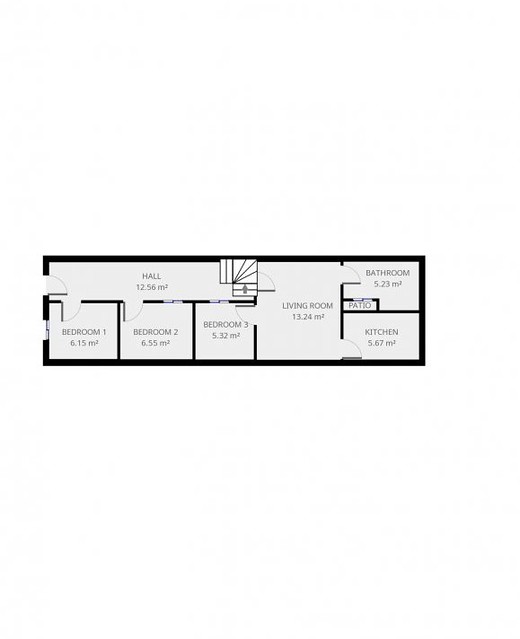This blueprint depicts an elongated, narrow structure resembling a mobile home. The floor plan is arranged longitudinally, with the right end featuring a bathroom positioned in the upper corner. Adjacent to the bathroom, there's a staircase leading to what appears to be a patio. Directly beneath the bathroom, in the bottom right corner, lies the kitchen. Moving left from the kitchen, the layout transitions into a more spacious area designated as the living room.

Further to the left, the blueprint outlines a sequence of three bedrooms labeled Bedroom 3, Bedroom 2, and Bedroom 1. Above the bedrooms runs a hallway that spans the length of the home. At the leftmost end of the hallway, a square area with blinds is visible, accompanied by several undefined rectangular shapes, which likely serve as storage spaces, though their exact function is unspecified due to the absence of a key for the blueprints. Notably, in the upper right corner of the bathroom, a small rectangle is intriguingly labeled as a patio, adding an unusual element to the design.